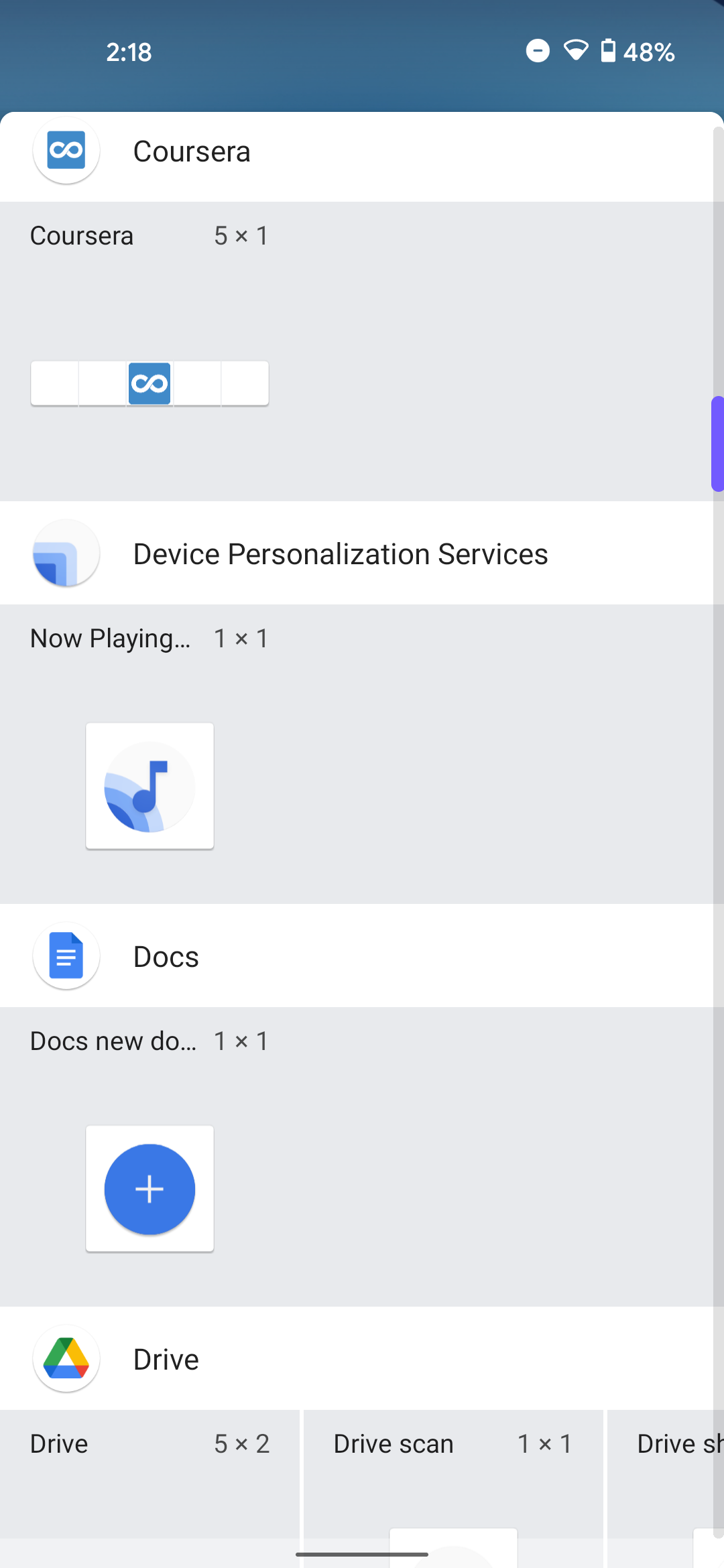This is a detailed mobile phone screenshot of an Android device, likely a Google Pixel based on the top-line font and the icons shown, though it could be any Android phone with custom fonts. The time displayed is 2:18, with both Do Not Disturb and Wi-Fi enabled. The Wi-Fi signal is weak, and the phone's battery is at 48% charge.

The screenshot displays a Google Drive account with various files. The first file is named "Corsair 5x1," followed by "Device personalization services now playing 1x1," "Docs," "Docs new document 1x1," "Google Drive," "Drive 5x2," "Drive scan 1x1," and "Drive SH," although the last file name is cut off.

There are multiple scroll bars visible, suggesting that this is an edited screenshot comprised of three different segments of the page, pieced together to appear as one continuous page. This editing process has resulted in some unusual artifacts, and the screen seems about one-third longer than it would be on a standard mobile device.